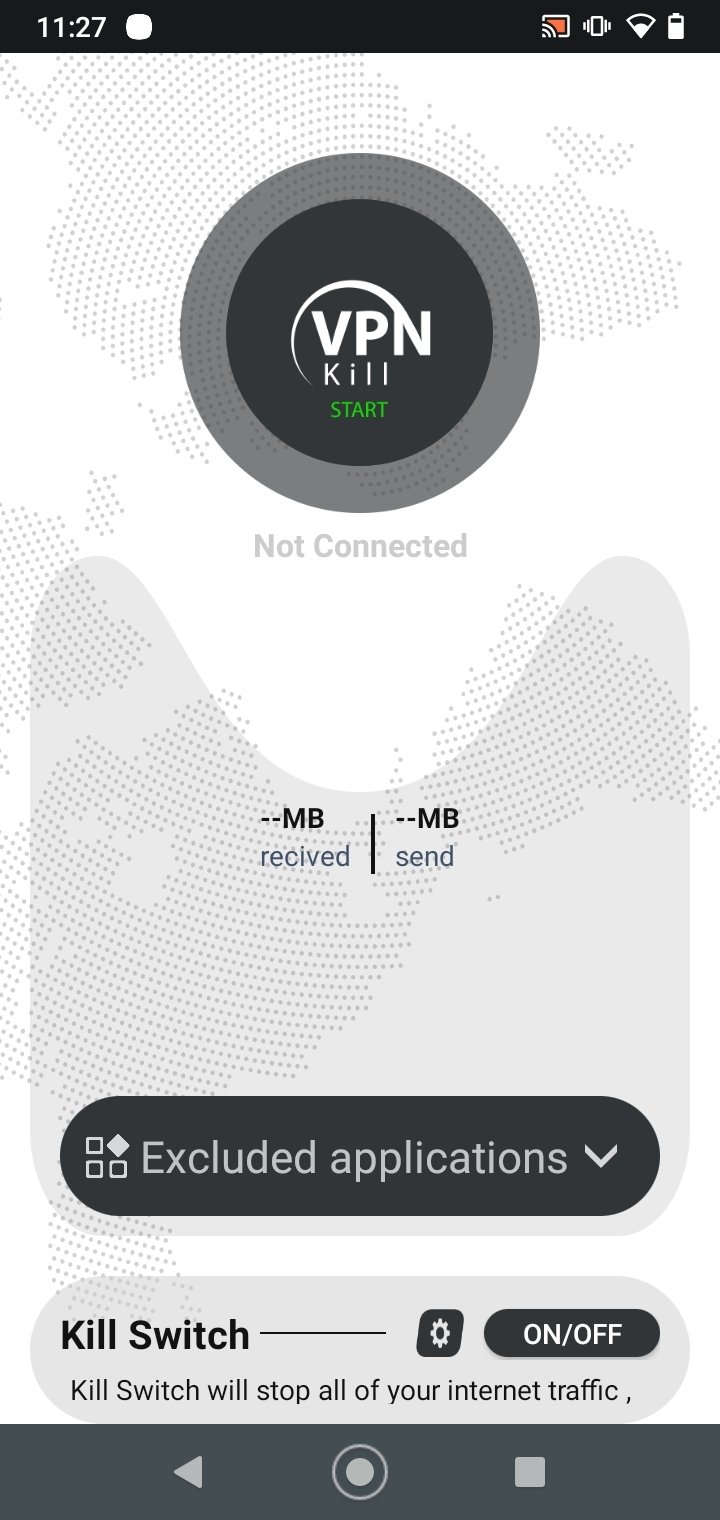The image depicts a mobile screen showing a VPN application interface. 

At the top of the screen, there is a black status bar. On the left, the time is displayed in white text as "11:27," followed by an icon resembling a square with rounded corners. On the right side of the status bar, there are multiple icons indicating the TV casting status (with a small orange mark inside), vibration mode, Wi-Fi signal strength, and battery level.

Beneath the status bar, the screen has a whitish background speckled with grey dots. In the center, there is a large grey circle with a black circle inside it. Inside the black circle, "VPN Kill" is written in white text, with the word "start" in orange text below it. Underneath this circle, "Not connected" is displayed in grey text.

Further down the screen, there are two black dashes accompanied by "MB received" and a black line, followed by "MB sent" with two additional black dashes.

Below this information, there is a darker grey rectangular area containing white text that reads "Excluded Applications" with a down arrow to the right. To the left of this text, there are three squares and a diamond shape that appears to be filled in.

At the bottom of the screen, a section in black displays the text "Kill Switch," followed by a line, a gear icon, an on/off toggle switch, and the description "Kill switch will stop all your internet traffic."

Finally, the bottommost part of the screen has a grey bar featuring a left-pointing grey arrow, a record symbol in the center, and a stop or square icon on the right.